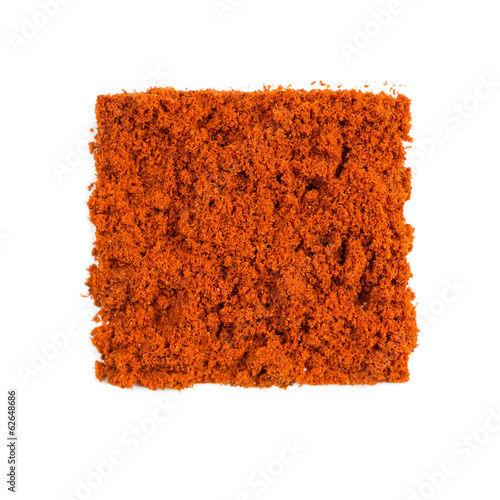The image features a rust-colored, porous, and spongy square-shaped material positioned against a clean white background. The material has an orange-brown hue and resembles a cluster of small particles or crumbs, with some bits flaking off the top, creating an irregular edge. The texture appears somewhat similar to brown sugar or a powdery substance, with small gaps throughout the mass revealing darker areas within. Diagonally faint in the background, the words "Adobe Stock" are visible, indicating this is a stock photo. Vertically aligned text in the lower left-hand corner reads "Adobe Stock 62648686" in small black font.